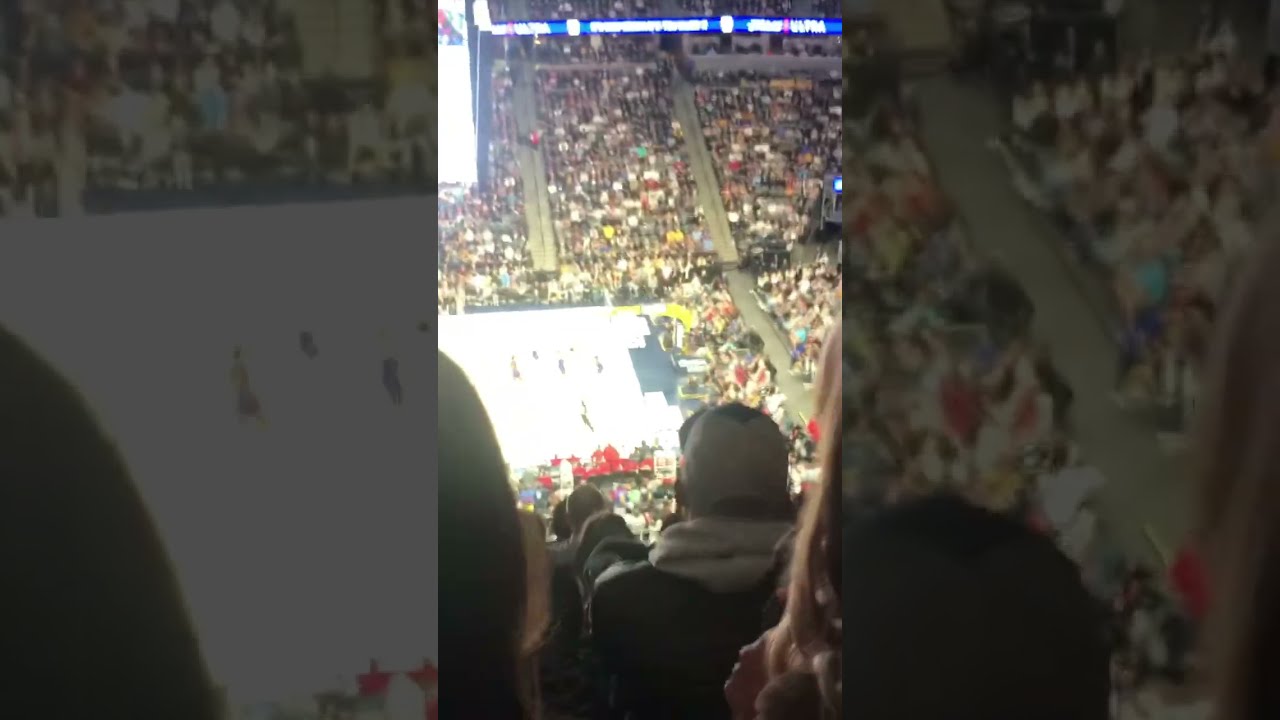The image captures a hockey game from the vantage point of a high seat in the stands, possibly the nosebleed section. The expansive, bright arena appears predominantly white due to the intense camera flash, which obscures the details of the court and player uniforms, leaving only faint specks of color to signify the few visible players. The arena is filled with layers upon layers of enthusiastic fans, emphasizing its large, professional scale. In the foreground, a man wearing a ball cap, jacket, and hooded sweatshirt is prominent, along with another indistinct figure beside him. A jumbotron in the top left corner of the image is also lit up brightly, contributing to the overall brightness, and a blue banner with the words "Bloody Stuff" in white can be seen. The meticulous details of the crowd, the bright lighting, and the high perspective collectively give a sense of the enormity and vibrant atmosphere of the event.